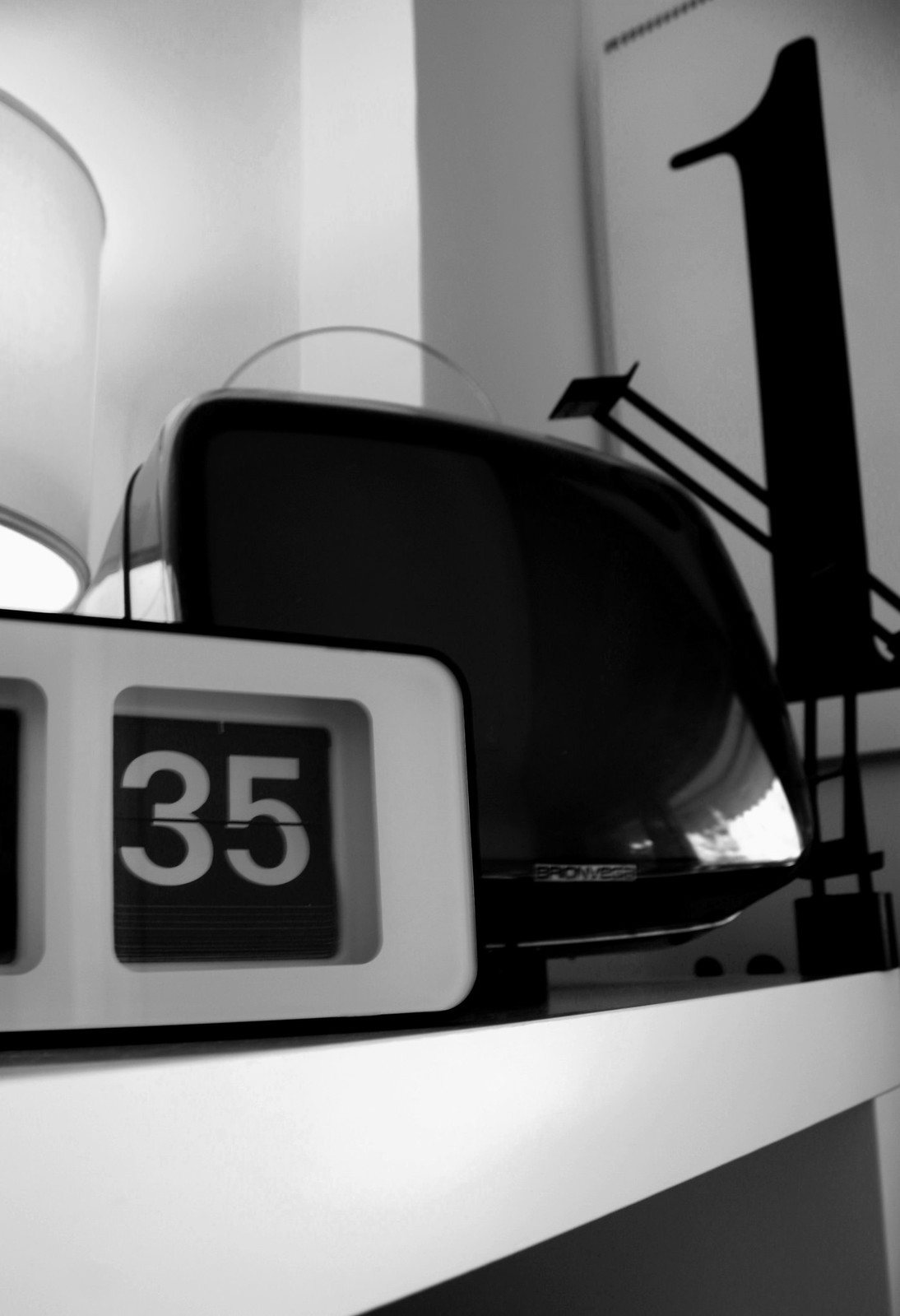This detailed close-up photo showcases an alarm clock positioned on a white table, suggesting it could be in either a bedroom or an office space. Only part of the clock is visible, focusing on the minute display which currently reads 35. The time is displayed in white numbers on a black background. The clock’s exterior appears to be predominantly white, contrasting with what seems to be a black body. Adjacent to the clock is a black screen, possibly a computer monitor. To the right of this setup, there is a large black "1" set against white curtains. The room’s walls are all white, and the ambient lighting emanates from a lamp.